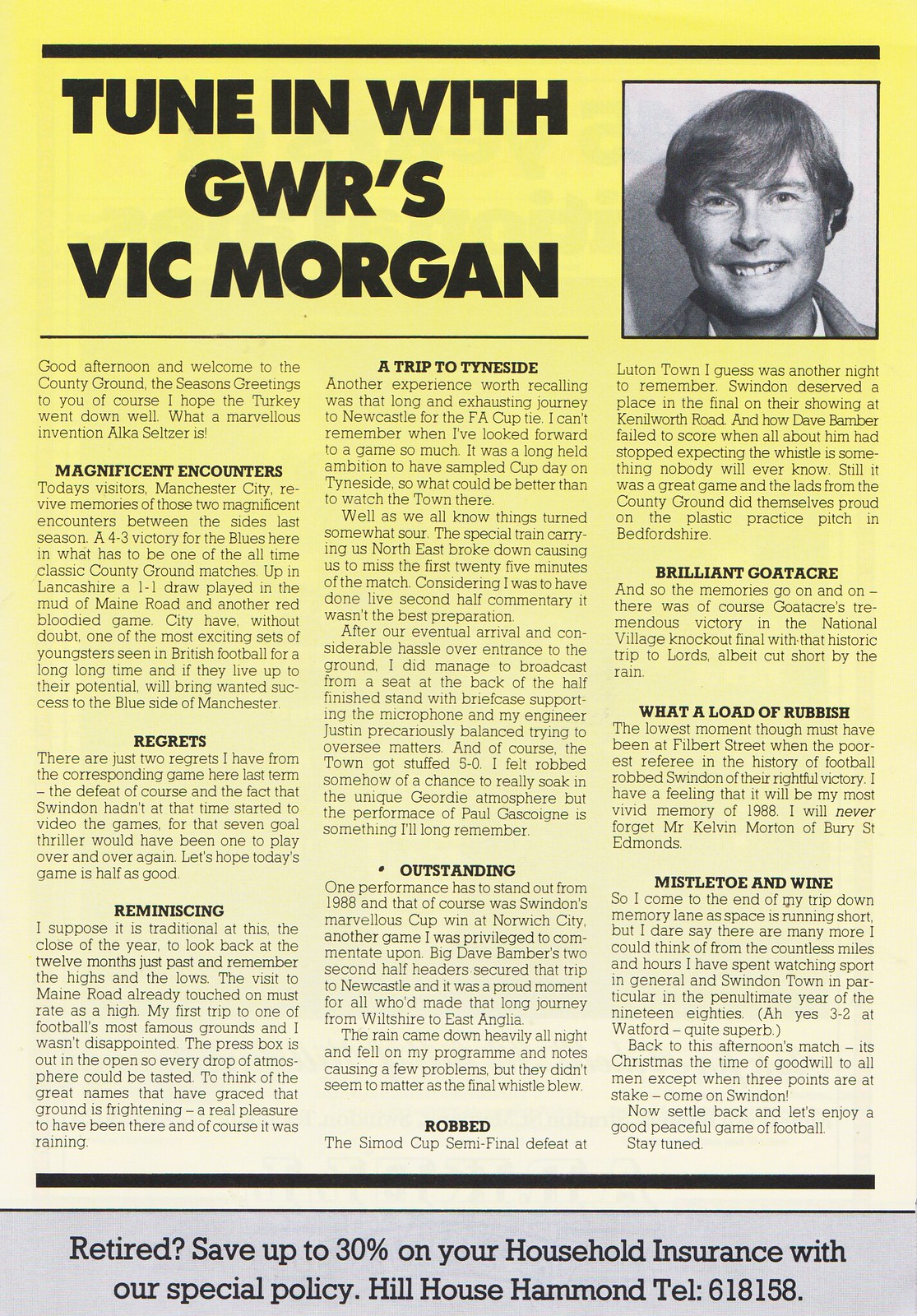This image is a page from a newspaper or magazine with a predominantly yellow background. At the very top, in black print, the title reads, "Tune in with GWR's Vic Morgan." To the right of the title, there is a small black-and-white photograph of Vic Morgan, smiling and looking directly at the camera, with his hair styled over his forehead. The main body of the page is divided into several columns, each containing articles written by Vic Morgan. The columns are titled "Magnificent Encounters," "Regrets," "Reminiscing," "A Trip to Tyneside," "Outstanding," "Robbed," "Brilliant Goatacre," "What a Load of Rubbish," and "Mistletoe and Wine." These titles hint at various themes, possibly reflections or commentary, likely related to soccer, as indicated by phrases like "welcome to the country ground." At the very bottom of the page, there is an advertisement with a gray border reading, "Retired? Save up to 30% on your household insurance with our special policy, Hill House Hammond. Telephone 618-158."